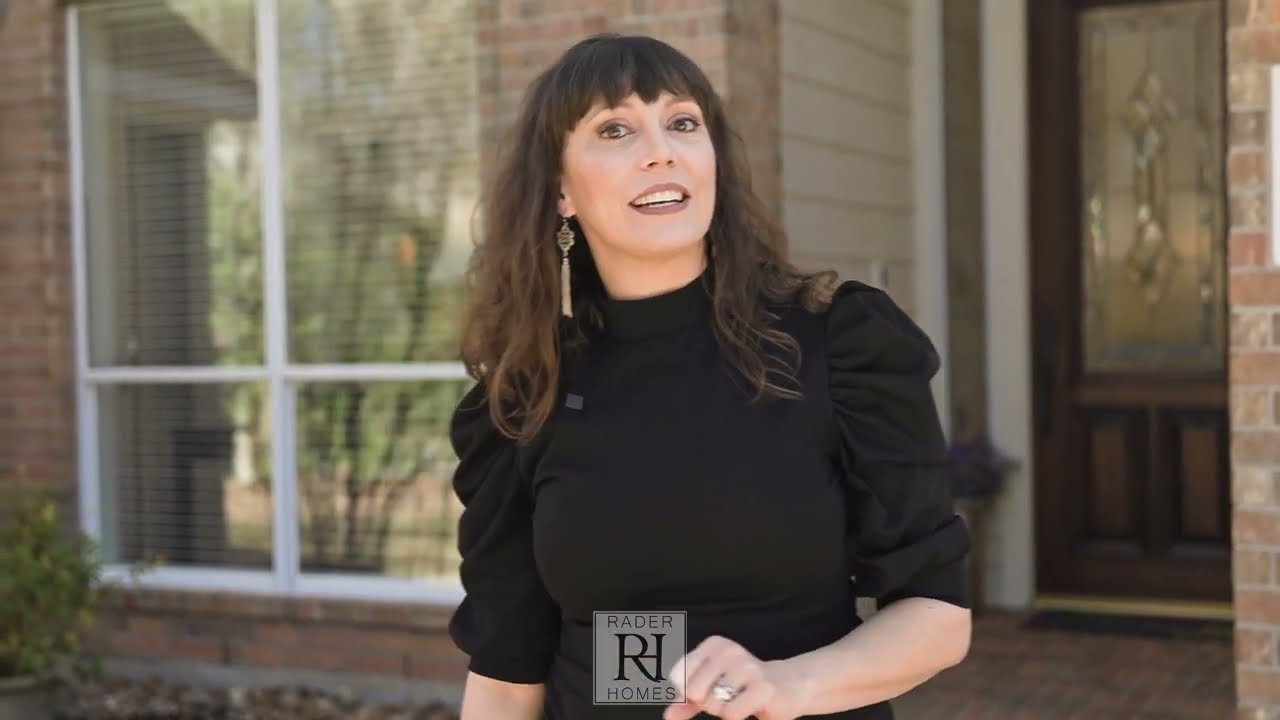The photograph features an attractive young woman in her late 20s to early 30s, standing outside in front of a brick house. She has long, straight brown hair with bangs, cascading softly over her shoulders. Her complexion is fair, and she wears makeup, accentuating her smiling face. Her head tilts slightly upward, and her gaze is directed a little off to the side.

She is dressed in a black outfit with puffy three-quarter length sleeves, which could be a top or a dress. She wears long, gold drop earrings that start with a round piece at the top and extend down to a dangling part. On her left hand, rings are visible, including a possible wedding ring, while her right arm hangs straight down by her side.

In front of her, around belly level, an image is projected onto her, displaying a logo with the words "Raider Homes" and an overlapping "RH" in the center. The scene behind her includes a front door of dark wood with an etched tall window, a large picture window with large panes at the top portion and smaller panes at the bottom, and a brick area to the left. A planter with greenery is visible in the bottom left corner of the image.